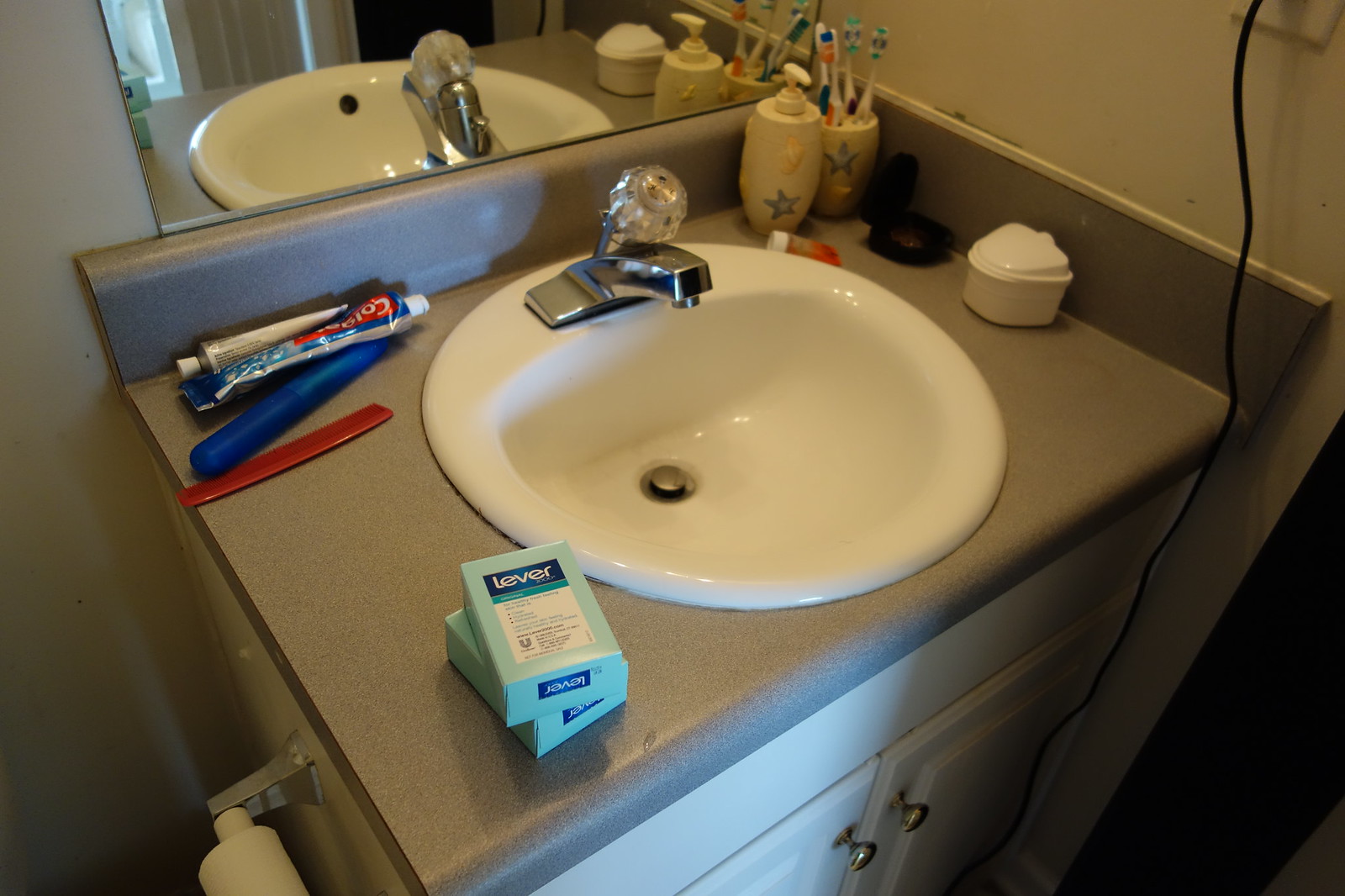A standard porcelain white bathroom sink is the focal point of the image, featuring a silver faucet. In the upper left corner, you can spot some toothpaste. Adjacent to it, there are two toothbrushes and a couple of soap containers labeled "Lever." Although the exact details are unclear, they might be soap bars. To the right of the sink, three more toothbrushes rest in a white container adorned with a star. Next to this, a matching white soap dispenser, also embellished with a star, sits beside a black retainer case and a white retainer case. The background includes a black plug in the wall, gray countertops, and white cabinet doors. The photo captures a typical, everyday bathroom sink setup.